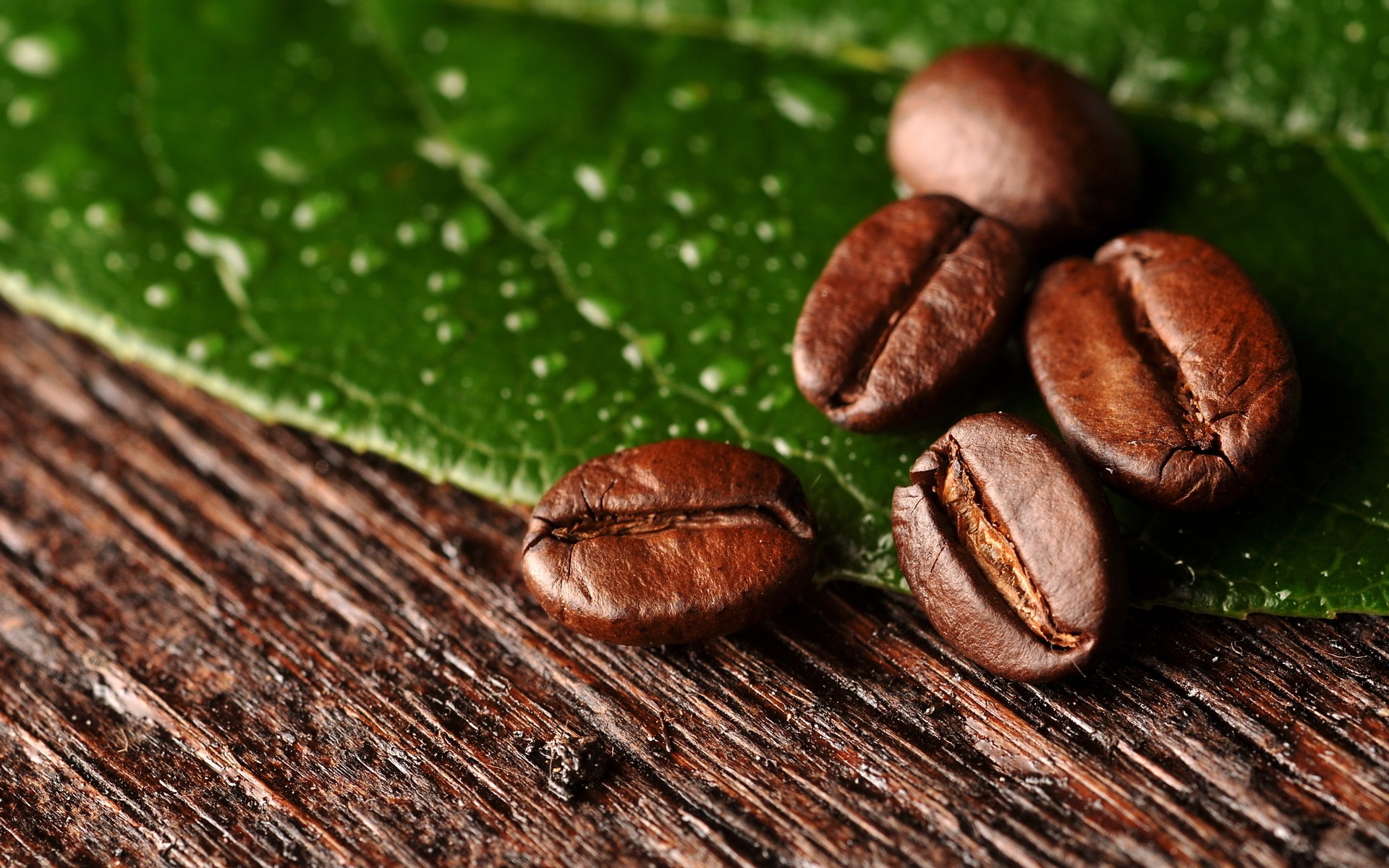A close-up photograph in landscape mode showcases five dark brown coffee beans with a distinctive stripe running down the middle. The image is sharply focused on the coffee beans, revealing their light brown centers. The beans are positioned on a rough, dark brown wooden surface that displays noticeable cuts and indentations, suggesting it's unpolished and natural. On top of the wood lies a dark green, leaf with a light yellow trim, adorned with droplets of water or dew. The leaf, which extends to the top of the image, is slightly out of focus to emphasize the coffee beans. Among the five coffee beans, three rest completely on the leaf, while two are partially hanging off it, with one more prominently on the wood surface. The primary colors in this detailed composition are brown and green, highlighting the rustic and natural setting.